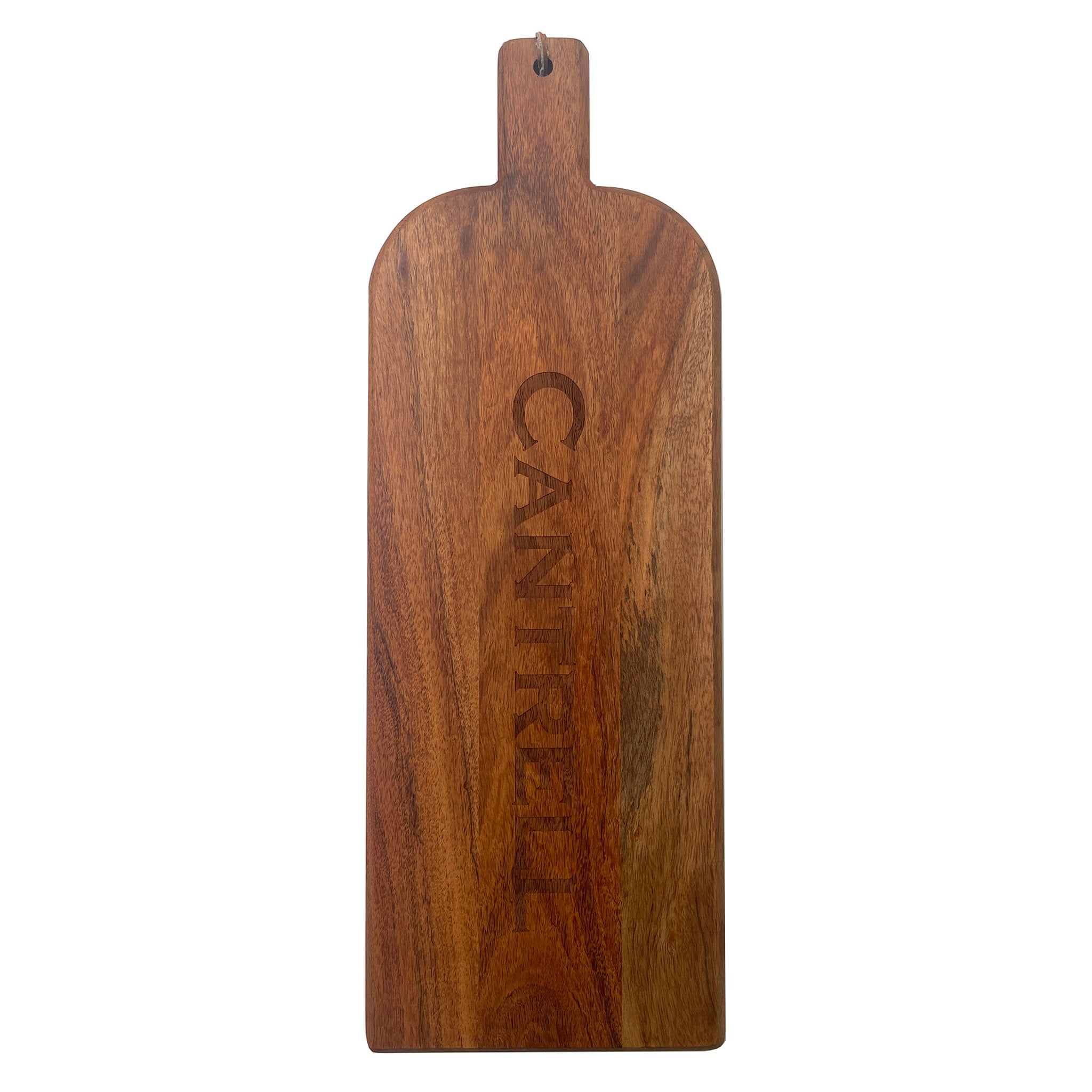In the image, we see a cutting board made of dark brown wood with varying shades of lighter and medium brown patterns throughout. The board is shaped somewhat like a wine bottle, featuring a handle at the top with gently curved sides that taper into a flat bottom. There is a hole in the handle, through which a piece of string or leather is threaded. The board appears textured with visible grains and knots, accentuating its rustic appeal. Engraved vertically in darker brown lettering across the center of the board is the word "Cantrell." The cutting board is displayed against a plain white background, making the textures and colors of the wood stand out prominently. The entire design has an old-fashioned, well-worn aesthetic, suggesting it may be a personalized item.